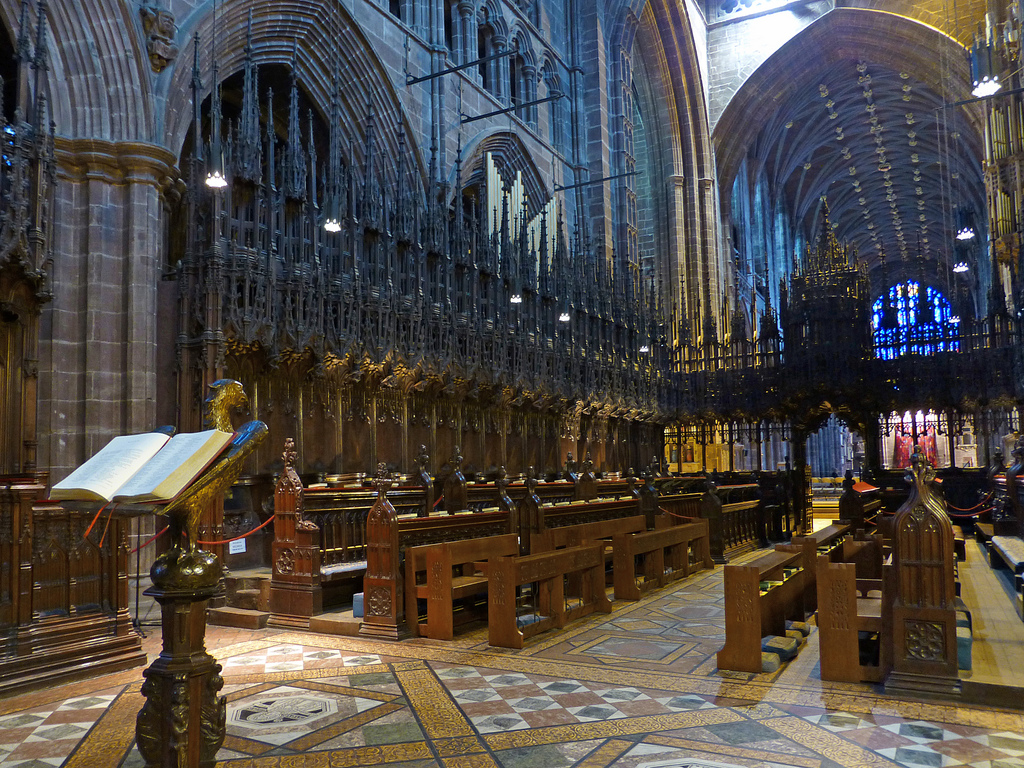The photograph captures the intricate interior of a Gothic cathedral, reminiscent of Notre Dame, characterized by its soaring arches and iron embellishments. The foreground prominently features an ornately decorated wooden lectern, crafted in the shape of a large bird with an open Bible resting atop its wings, held in place by a red bookmark. The lectern is situated on the left side of the image, facing out over the chapel. The middle ground is filled with dark brown, carved wooden pews arranged diagonally, each equipped with kneeling rails, indicating its use for Catholic worship. Between the pews, intricately decorated wooden fencing adds to the cathedral's rich interior. The cathedral's walls are constructed from medium gray stone, adorned with ironwork that rises into pointed arches. The soaring ceilings boast ornate lighting fixtures, while the floor is a mosaic of gold, red, and various shades of gray tiles. Towards the back of the cathedral, a red curtain and bright lighting can be seen, adding depth to the majestic scene.